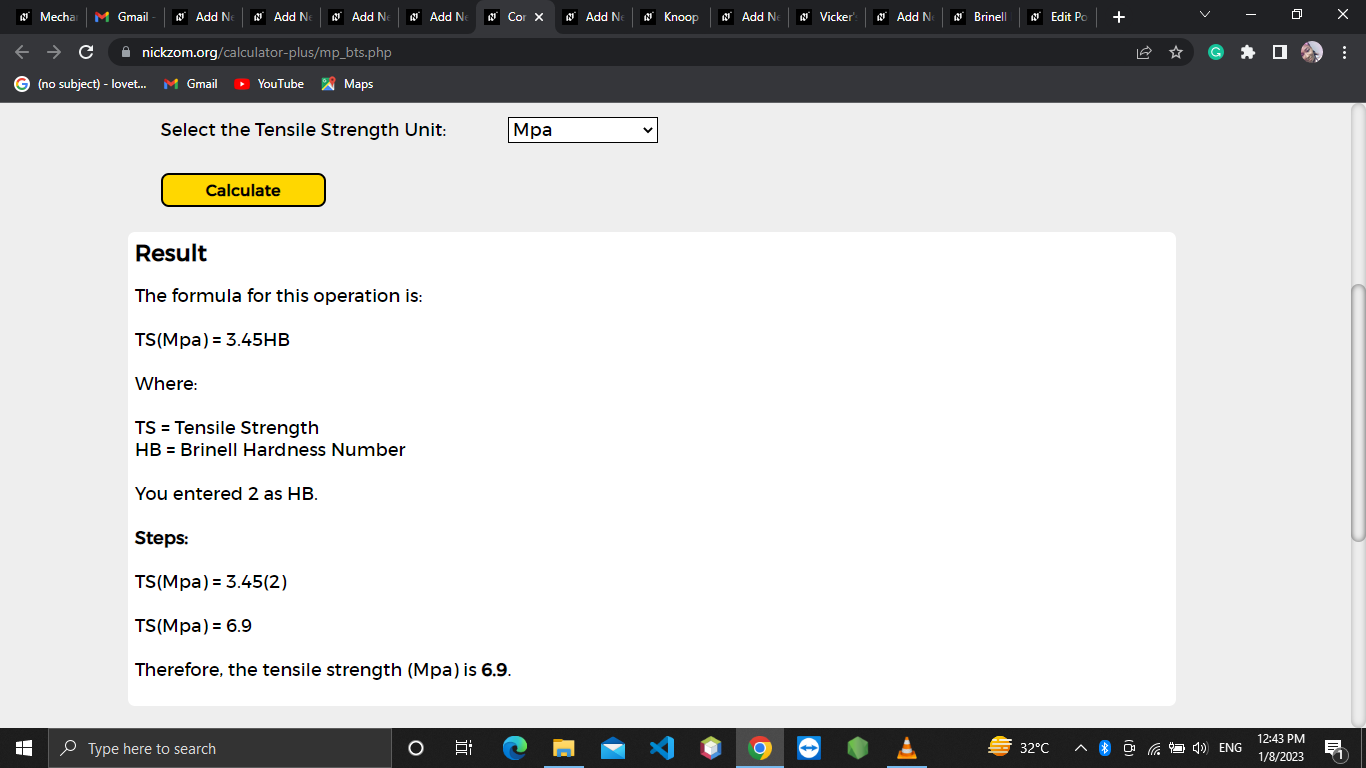A screenshot of a Windows 10 desktop featuring Google Chrome with an overwhelming number of open tabs, suggesting potential performance issues due to excessive memory usage. The address bar displays an unspecified URL, and the page is not bookmarked, as indicated by the unhighlighted star icon. The user seems to be navigating through Gmail, as inferred from the interface elements.

Central to the screenshot is a webpage with a technical form, likely for calculating tensile strength. The form, set against a gray background, includes black text prompts such as "Select the tensile strength unit," followed by "MPA" entered into a white input box. Below this, a yellow button labeled "Calculate" appears. Further instructions in black text within a white box read: "Resolve the formula of this operation is TS (MPA) = 3.5 HB, where TH = strength test and BH = Brinell hardness number. You enter 2 as BH steps. TS (MPA) = 3.5 (2). Therefore, the tensile strength of MBA is 6.9."

The taskbar at the bottom of the screen shows the Windows logo on the left and a search bar with "Type here to search." The taskbar icons are colorful, with elements in blue, yellow, green, and black. The timestamp on the screenshot is 12:48 PM, dated either January 8th or August 1st, 2023, denoted as 8/23.